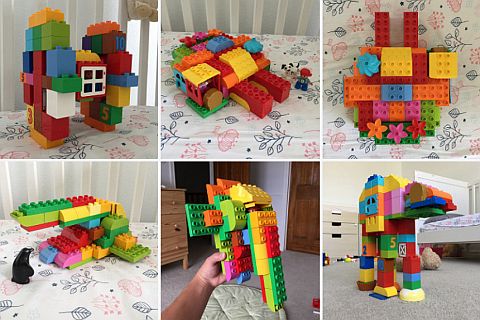This collage showcases six vibrant photographs of various Duplo Lego creations, each image separated by a thin white border. The Lego designs are laid out on a patterned tablecloth predominantly featuring white with a flowery or leaf motif. In the upper left image, there's a multi-colored house-like structure with yellow, green, blue, orange, and a distinctive white window, flanked by two pillars. Adjacent to this, in the middle top, is another house design laid out on the patterned tablecloth. The bottom right image captures an imaginative walking dinosaur crafted from the brightly colored Duplo bricks. Another thumbnail illustrates a robot-like figure, and scattered among the remaining images are unique constructions including what appears to be a camel. The compositions brilliantly use a spectrum of colors such as light green, yellow, orange, and red to bring these imaginative figures to life.